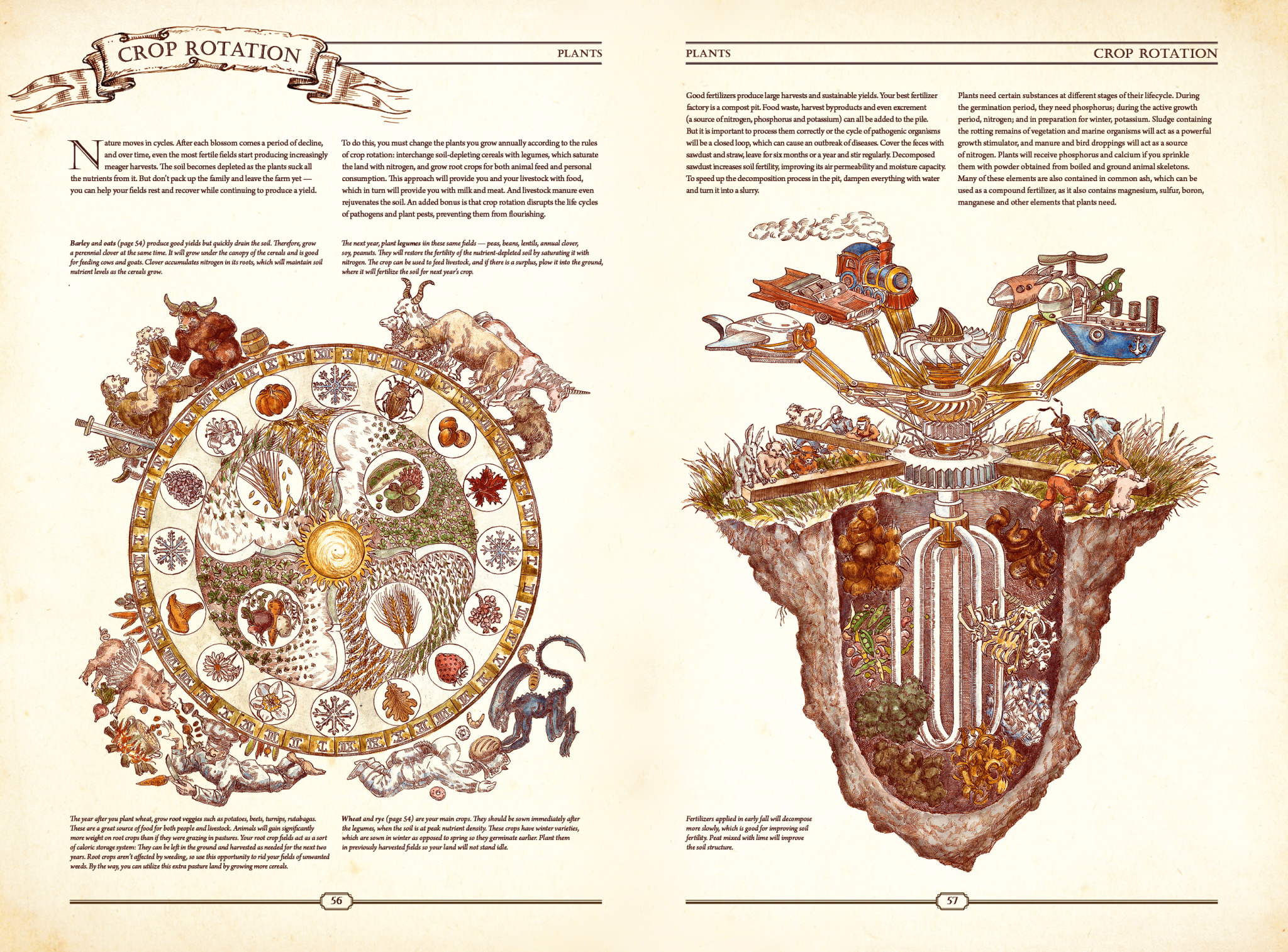The side-by-side images share a light cream-colored background and feature detailed headers, informative text, and illustrative drawings. 

**Left Image: Crop Rotation Plants**
The left image, titled "Crop Rotation Plants," provides an insightful explanation regarding the natural cycles in agriculture. It discusses how, after each blooming phase, there's a subsequent period of decline where even the most fertile fields suffer from nutrient depletion. This happens because plants continuously extract essential nutrients from the soil. However, it advises not to abandon the farm but instead to let the fields rest and recover while still maintaining productivity. The illustration in the center of this image depicts a circular diagram featuring seasonal elements such as bugs, leaves, and snowflakes, symbolizing the changing seasons and the continuous cycle of nature.

**Right Image: Effective Fertilizers**
The right image focuses on the significance of good fertilizers in producing large harvests and stable crops. It introduces the concept of a compost pit as the best source of organic fertilizer, emphasizing the addition of food waste, harvest byproducts, and excrement to create nutrient-rich compost. The accompanying illustration shows a compost pit with a mechanism for turning the compost, visually explaining the process. Additionally, the drawing features boats, planes, and airplanes on a circular loop emerging from the ground, possibly hinting at the interconnectedness and global importance of sustainable farming practices.